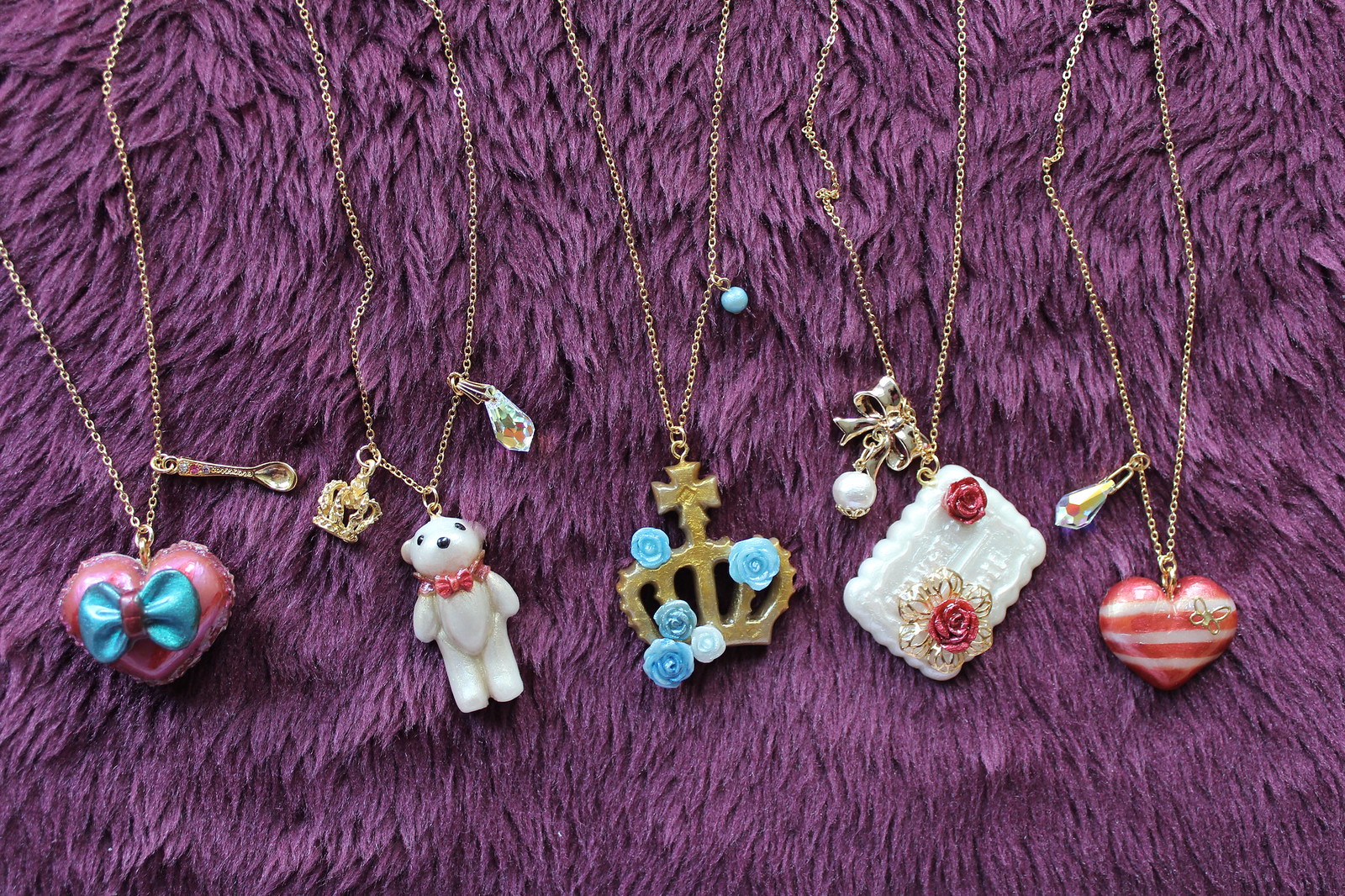This photograph showcases a collection of five gold-toned chain necklaces, each adorned with unique pendants, placed on a shaggy purple surface. From left to right, the first necklace features a pink heart locket with a turquoise bow, complemented by a small gold spoon charm on the chain. The second necklace exhibits a white teddy bear with a red bow tie, a gold crown, and an additional crystal pendant. The third necklace displays a regal gold crown crowned with a cross, adorned with four blue roses and one white rose, coupled with a small blue bead on the chain. The fourth piece is a square pendant resembling a birthday cake, decorated with two red roses, gold-toned leaves, and a small bow with a pearl-like charm. The final necklace presents a red and white striped heart locket with a butterfly in the right-hand corner and a crystal charm similar to the one on the teddy bear necklace, hanging from the chain.